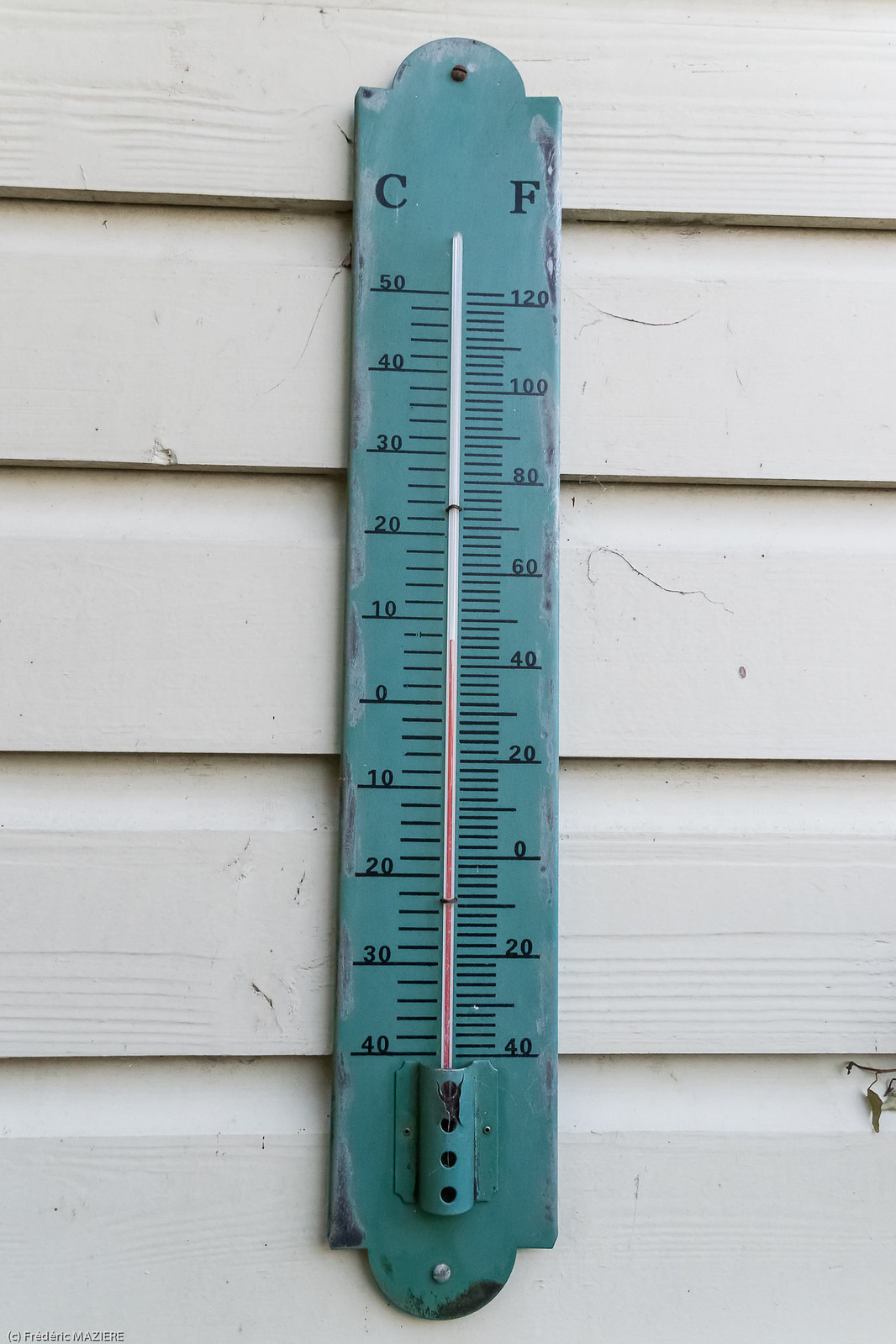The photograph depicts an outdoor metal thermometer attached to a wooden siding wall. The thermometer, painted green, displays temperature readings in both Celsius and Fahrenheit. The current temperature reads approximately 46 degrees Fahrenheit, which is just under 9 degrees Celsius. The thermometer is affixed to the wall with screws, and the top screw shows significant rust, indicating prolonged exposure to the elements, while the bottom screw appears weathered but less corroded. The green paint on the thermometer is chipped along its edges, revealing rust, particularly around the bottom. The wooden siding, painted white, features either tongue-and-groove or overlapping boards, complementing the aged yet enduring look of the thermometer.